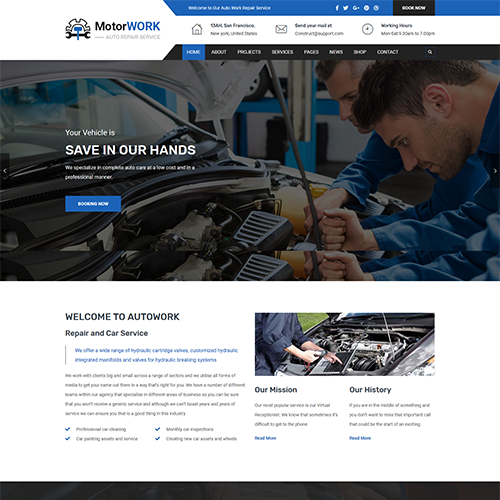The screenshot captures the homepage of the "Motorwork" website, which specializes in auto repair services. Dominated by a clean blue and white color scheme, the top part of the page features a blue banner overlaying a white one. The Motorwork logo, prominently displayed, consists of a gear icon with a hammer and a wrench crossed inside it, embodying the spirit of their repair service.

The headline on the webpage reads, "Your vehicle is safe in our hands. Welcome to Autowork Repair and Car Service." Underneath, the text begins to describe their offerings, mentioning a wide range of hydraulic cartridge services, although part of the text appears blurry. The navigation menu provides links to various sections including Home, About, Products, Services, Pages, News, Shop, and Contact, facilitating easy access to essential information.

Central to the homepage is an image of two technicians diligently working under the hood of a car, their actions obscured but indicative of focused maintenance work. Below this main image, another photo depicts a person working on a computer while also examining the engine of a car, suggesting a blend of digital diagnostics and hands-on repair expertise.